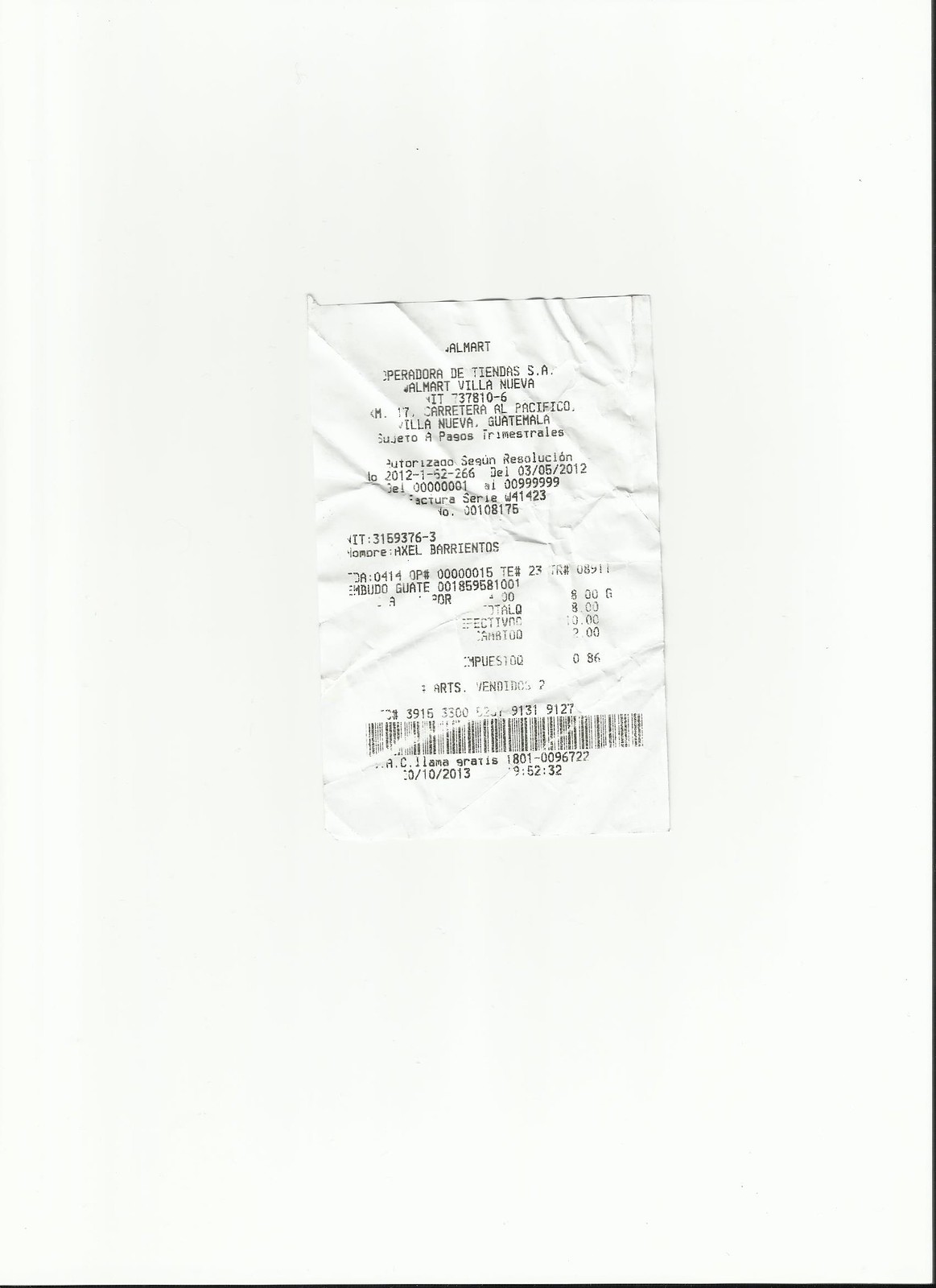The image features a photograph of a heavily wrinkled receipt placed at the center of a large, vertically oriented cream-colored rectangle. The rectangle is bordered by a thin black line on its bottom and right sides, while the top and left sides remain unbordered. The receipt, which is visibly crinkly, appears to be scanned and is somewhat difficult to read. At the top, the receipt prominently displays the word "Walmart," indicating its origin. The text following the header is entirely in Spanish, and it includes the address "Villa Nueva, Guatemala," confirming its point of issue. The receipt, evidencing a purchase of only one item, is dated October 10, 2013, and bears a barcode at the bottom.